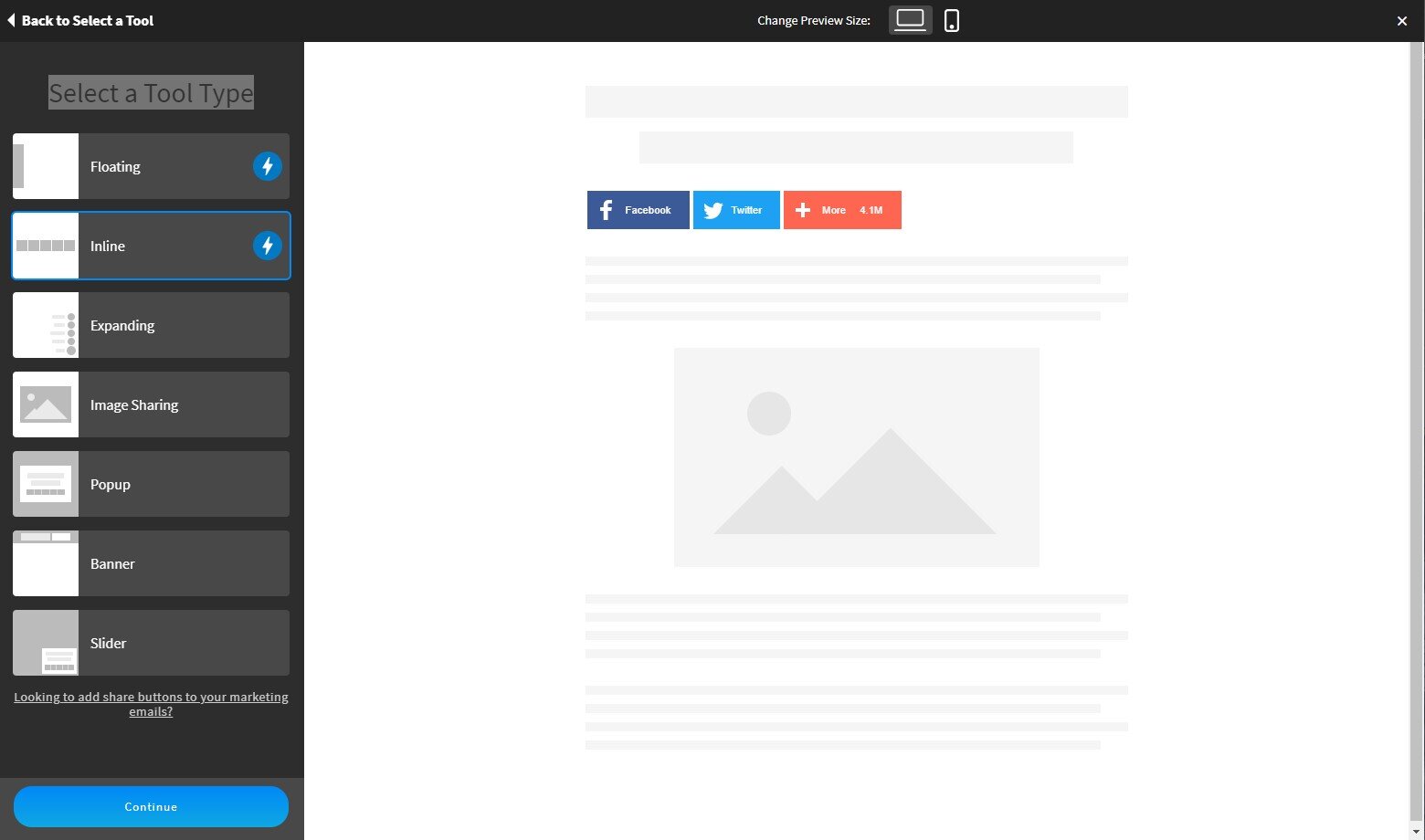Screenshot of a Website Interface for Social Media Sharing Tools:

In the top left corner of the interface, there's a label that reads "Back to Selected Tool." Directly below this, another label displays "Selected Tool Type." The interface adopts a nocturnal theme with black text on a gray background, giving it a distinctive look.

Below these headings, a set of options is presented, including "Floating," "Inline" (which is currently selected), "Expanding," "Image Sharing," "Popup," "Banner," and "Slider." At the bottom of this tools section, a message inquires if users want to "Add Share Buttons to Your Marketing Emails."

Centered at the top, there is an option titled "Change Preview Size," accompanied by icons of a computer and a phone, suggesting the ability to preview the tool's appearance on different devices, which is a useful feature.

The main section of the page is minimalist, showcasing Facebook, Twitter, and a generic "More" button. The "More" button intriguingly includes a statistic of "4.1 million," though its context remains unclear.

In the bottom left corner, a prominent blue button labeled "Continue" indicates a sequential process, prompting users to proceed to the next step after making their selections.